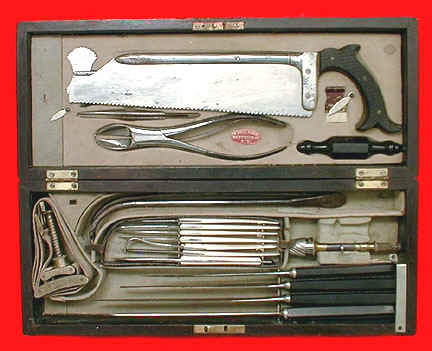This image depicts an opened black toolkit resting on a red cloth background. The kit, designed to fold shut with visible golden hinges and snap closures along the middle and edges, features an array of tools securely nestled in a gray, possibly Velcro-lined, interior. At the top, there is a substantial metal saw with a black curved handle and serrated blade, accompanied by a pair of metal pliers or clippers and a small black item in the lower right corner. The bottom half of the toolkit contains an assortment of multi-tools, including spiky implements, small screwdrivers, and picks, positioned in a neat arrangement. The overall setup suggests a comprehensive set of utensils and tools suitable for various precision tasks.